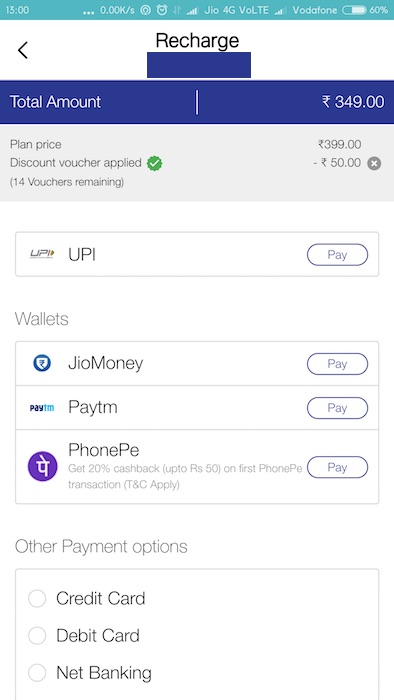The image displays a Vodafone recharge screen. At the top, a turquoise bar features various icons including Wi-Fi signal strength and a battery indicator at 60%. Below this bar, the screen is predominantly white with black text that reads "Recharge." 

On the left side of the screen, there is a navy blue horizontal rectangle. Adjacent to this is a section labeled "Total Amount" in a white-separated area, which displays $349. Beneath this is another section in a grayish rectangle that reads "Plan Price" with a value of $399 (currency symbol unclear). A discount voucher has been applied, indicated by a green check-marked Twitter symbol, reducing the amount by $50.

Further down, there is a section labeled "UPI" for payment options. Below, various wallet payment options are listed: JIO Money Pay, PAYTM Pay, PhonePe Pay. Additionally, other credit options include payments via credit card, debit card, or net banking.